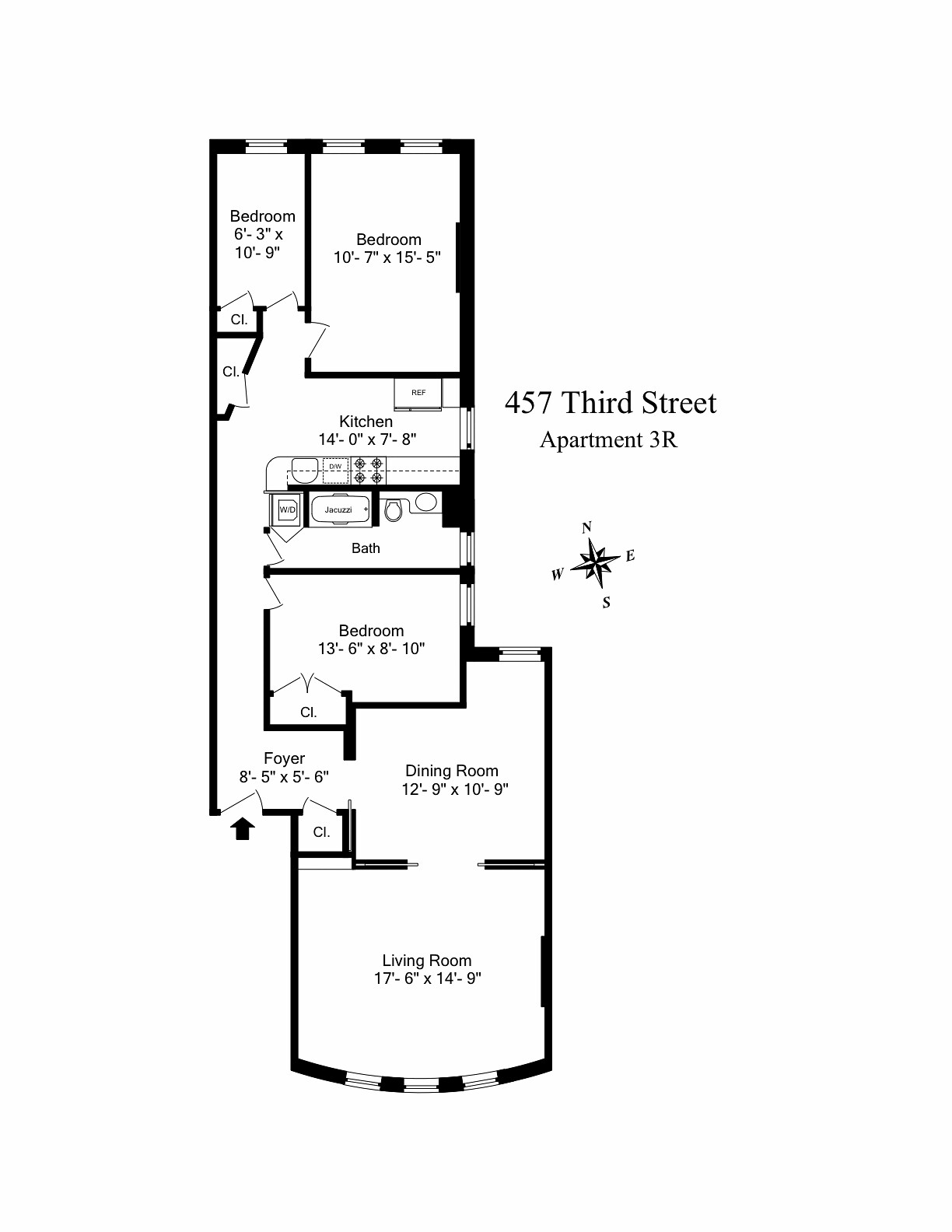This detailed blueprint outlines the layout of an apartment located at 457 3rd Street, Apartment 3R, accompanied by a compass symbol indicating Northeast and Southwest directions. The apartment features a master bedroom measuring 10'7" x 15'5" with an adjacent closet. There is a smaller bedroom at the top of the layout, measuring 6'3" x 10'9", also with a closet. 

The kitchen is generously sized at 14'0" x 7'8" and appears to be fully equipped with appliances. A hallway connects the kitchen to the dining room, passing by an undimensioned bathroom and a bedroom measuring 13'6" x 8'10" that includes a double-width closet.

Upon entering the apartment, there is a foyer measuring 8'5" x 5'6" with an accompanying closet. The dining room, measuring 12'9" x 10'9", sits near the spacious living room, which measures an impressive 17'6" x 14'9". This apartment, with its elongated layout, offers ample living space and storage options, presenting a well-thought-out design for potential residents to consider.